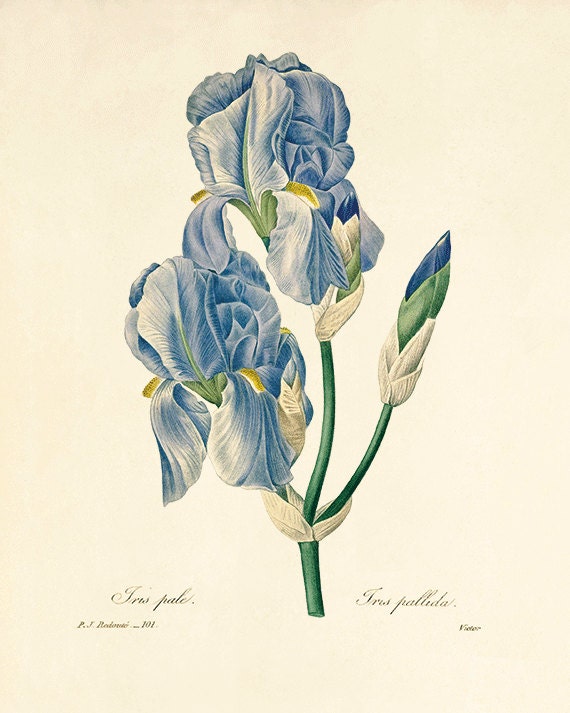This detailed drawing, possibly using colored pencils, depicts an iris flower with a vintage, scientific illustration style. The flower is centered on a parchment-colored paper background, emphasizing its aged appearance. The main stalk supports three stems: two fully bloomed flowers, showcasing pale blue and white petals with yellow accents, and a third, green stem with a small blue bud. Surrounding the flowers are a few green leaves. At the bottom, the text reads "iris pale" or perhaps "iris palida," along with additional smaller text. The names "Victor" and "P.J. Redonier" are inscribed on the left and right sides, respectively, hinting at possible artists or botanists. French text, including the word "trespasser," is also visible, adding a layer of intrigue to the artwork's origin or message.